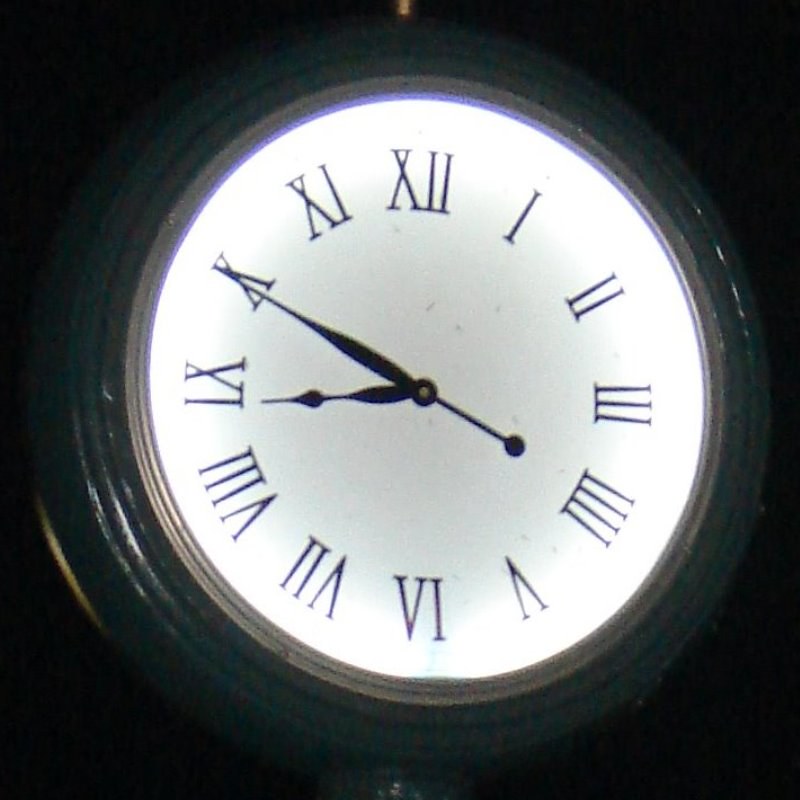In this image, we're looking directly at a large circular clock, likely designed for a public space such as a train station. The clock's prominent and smooth outer rim is dark grey or black metal, with little screws or rivets holding it in place. The clock face is illuminated, shining through a white backdrop, ensuring visibility even at night. The inner rim of the clock has a light blue hue, adding to its contrast. The hour, minute, and second hands are black, currently showing the time as 8:50, with the hour hand on IX and the minute hand on X. Roman numerals, rendered in black, mark the hours. The outer rim is green, possibly made of wood or metal, and the clock appears to be mounted on a pole with a projection matching the green rim in width and color. The background of the image is entirely black, which further highlights the illuminated clock, although the image is somewhat fuzzy overall.